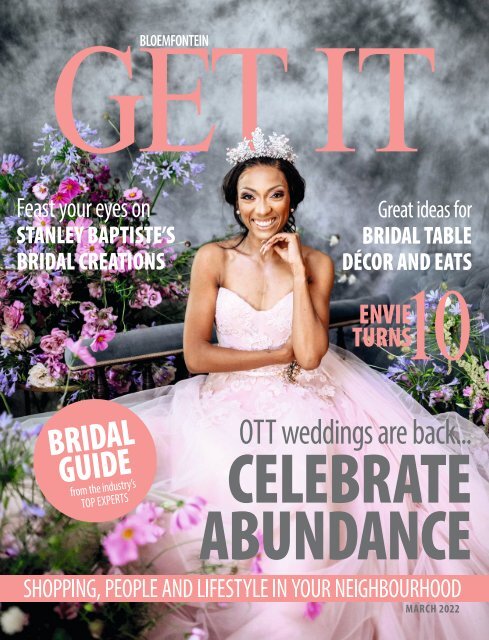This detailed magazine cover for the March 2022 issue of Blomfontein, titled "Get It," features a striking black-and-white misty background with vibrant pink, purple, and light blue floral arrangements. Central to the cover is an elegantly composed image of an African American model with long black hair swept away from her beaming face, adorned with a large tiara that appears to be either white or diamond-encrusted. She radiates joy with a broad smile and expressive eyes. The model is dressed in a pale pink, strapless wedding gown with a laced bodice and a voluminous mesh skirt, sitting demurely on a bench hidden by her dress. Text overlays the image, with small print at the top spelling out B-L-O-E-M-F-O-N-T-E-I-N, followed by large pink letters for GET IT. On the left, white text reads "Feast Your Eyes on Stanley Baptiste's Bridal Creations" and below it in pink, "Envie Turns Ten." On the right, it lists "Great Ideas for Bridal Table Decor and Eats" and in gray, "OTT Weddings Are Back. Celebrate Abundance." A pink circle with white text states, "Bridal Guide from the Industry's Top Experts." At the bottom, a pink strip highlights "Shopping, People, and Lifestyle in Your Neighborhood" in white letters, with "March 2022" in gray at the bottom right corner.